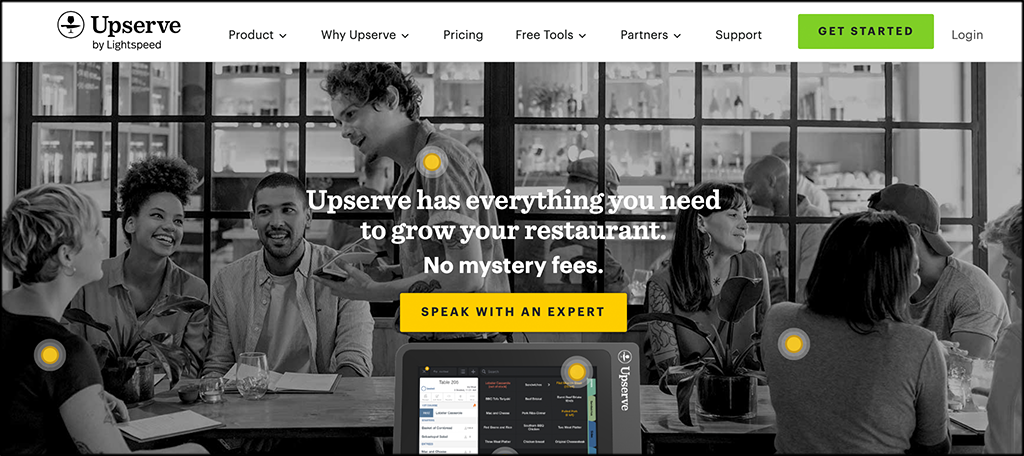The screenshot captures a webpage from "UpServe by Lightspeed." Dominating the upper portion of the screenshot is a prominent black rectangle, wider than it is tall. In the top left corner, it features the UpServe by Lightspeed logo, with a small circular emblem adjacent to it. The navigation menu spans across the top, presenting options such as "Product," "Why UpServe," "Pricing," "Free Tools," "Partners," and "Support." Alongside these, there is a green rectangular button labeled "Get Started" and an adjacent "Login" option.

Below the navigation bar, a grayscale image showcases a lively conference room scene with eight people seated around a table, all smiling and engaged in conversation. The backdrop features several large windows and three additional individuals visible behind them, seemingly associated with some product displays. The conference table itself is adorned with a houseplant, glasses, and notepads, contributing to a professional and yet inviting atmosphere.

Interspersed throughout the image are three yellow dots, each encircled, drawing attention to specific points. Centrally placed text within the screenshot proclaims, "UpServe has everything you need to grow your restaurant. No mystery fees." Beneath this statement, a prominent yellow button invites users to "Speak with an Expert." Further down, partially visible, appears to be a phone screen interface, possibly hinting at a mobile-friendly functionality or additional features.